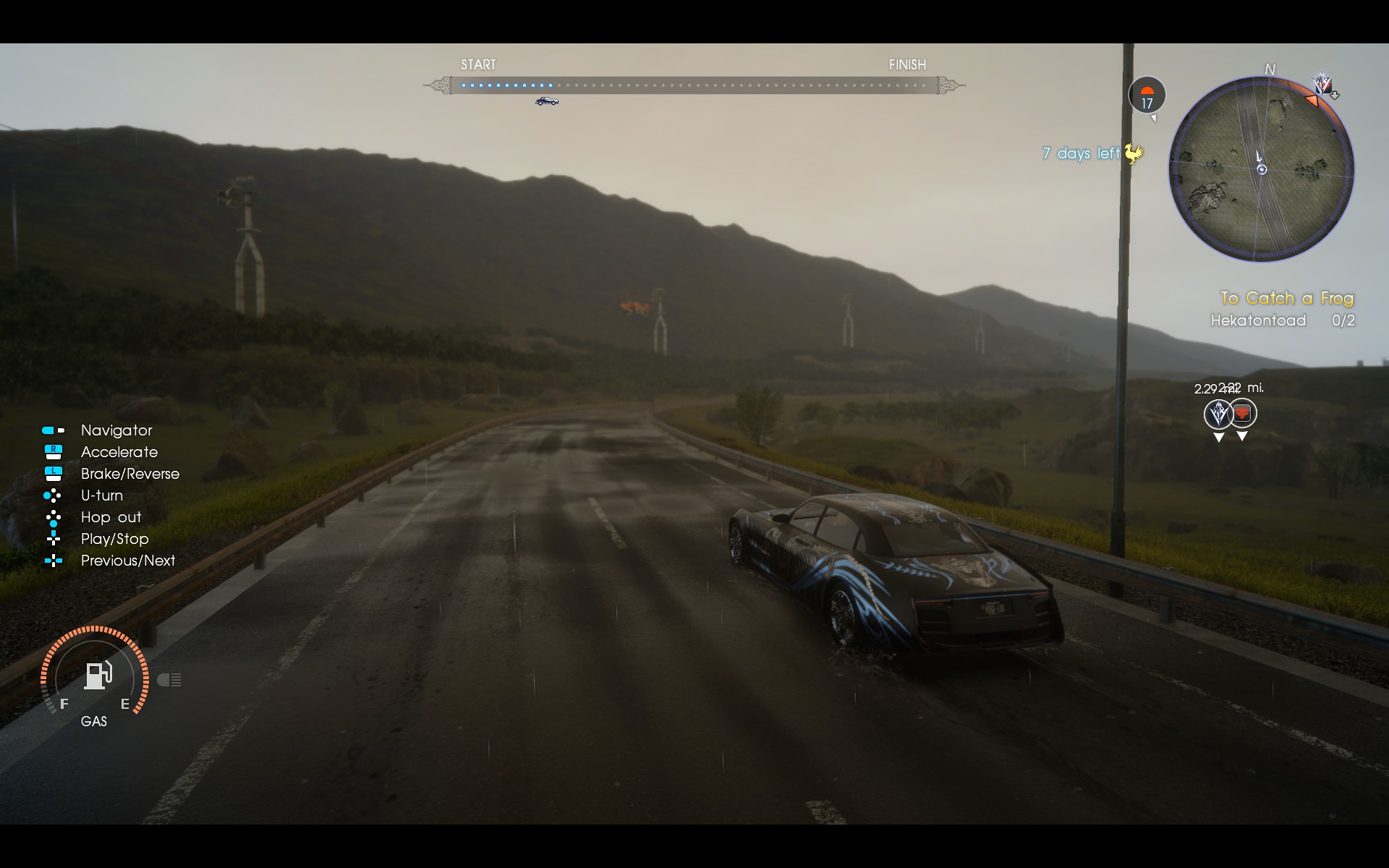In this dynamic video game scene, cars are racing through a picturesque countryside, flanked by towering structures that might be observation towers. The expansive landscape in the distance is dominated by large, rugged mountains. The game's user interface is populated with various buttons on the side, instructing players on how to navigate or accelerate, among other functions. A fuel gauge indicates that the tank is nearly three-quarters full. At the top of the screen, a tracking device likely displays the race's progress, showing the players' positions along the raceway, currently about one-third complete. Beneath this tracker, a helicopter hovers, perhaps serving as a race observer. A distinctive black car with blue markings is visible to the right of the player’s viewpoint, cruising along a two-lane highway marked by clear pavement lines. The road appears dark and potentially slick, hinting at recent rain, although no rain is currently falling.